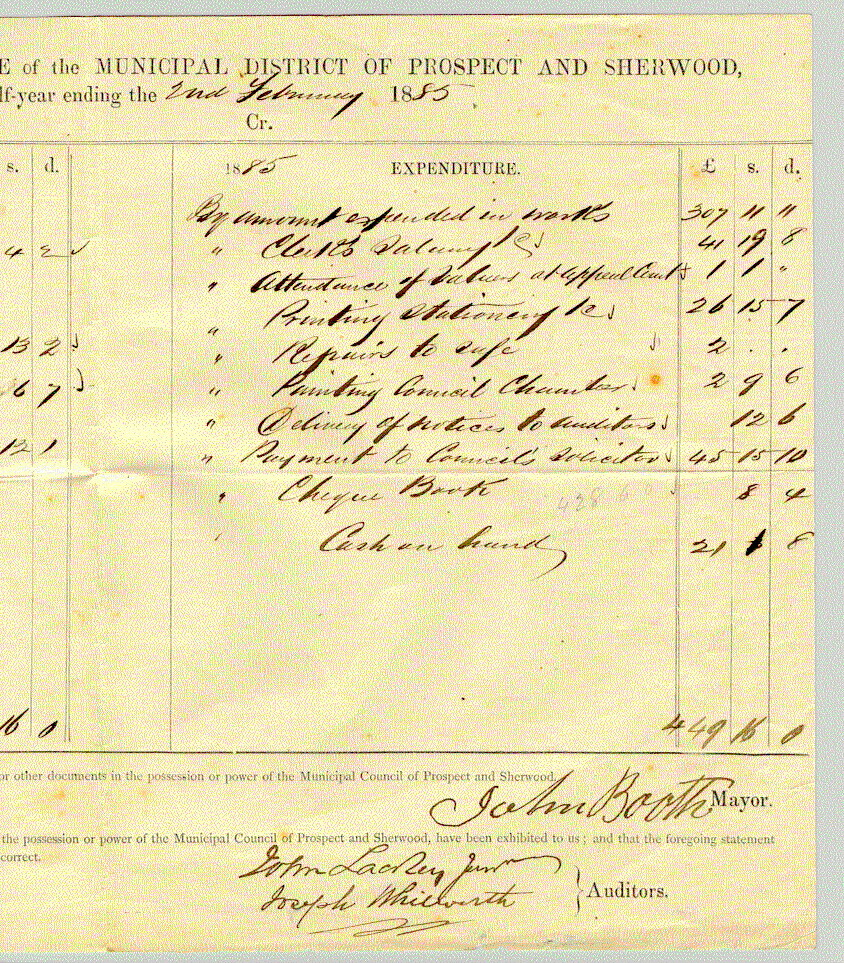The image depicts a yellowed, aged document from the Municipal District of Prospect and Sherwood. This piece of paper, dated from the year 1885, specifically references the half-year ending on February 2, 1885. It's an official government document with an authentic feel due to its heavy cursive handwriting, dark ink, and visible fold crease in the middle, suggesting it has been stored for a long time.

At the top of the document, in black type, it reads “Municipal District of Prospect and Sherwood.” The document details financial expenditures, as indicated by the large central column titled "1885 Expenditure." Listed items include “Printing,” “Stationery,” and “Repairs to Cafe,” with corresponding handwritten amounts in adjacent columns. These columns are organized with labels such as "S" and "D" on the left and three columns on the right for the totals, denoted by pound (£), shillings (S), and pence (D) symbols.

Handwritten signatures, including that of John Booth, who was the Mayor, appear along the bottom, signifying official approval. Additionally, there are signatures from auditors who verified the document. This intricate, handwritten document, laden with numbers and cursive notations, provides a fascinating glimpse into governmental financial records from the late 19th century.